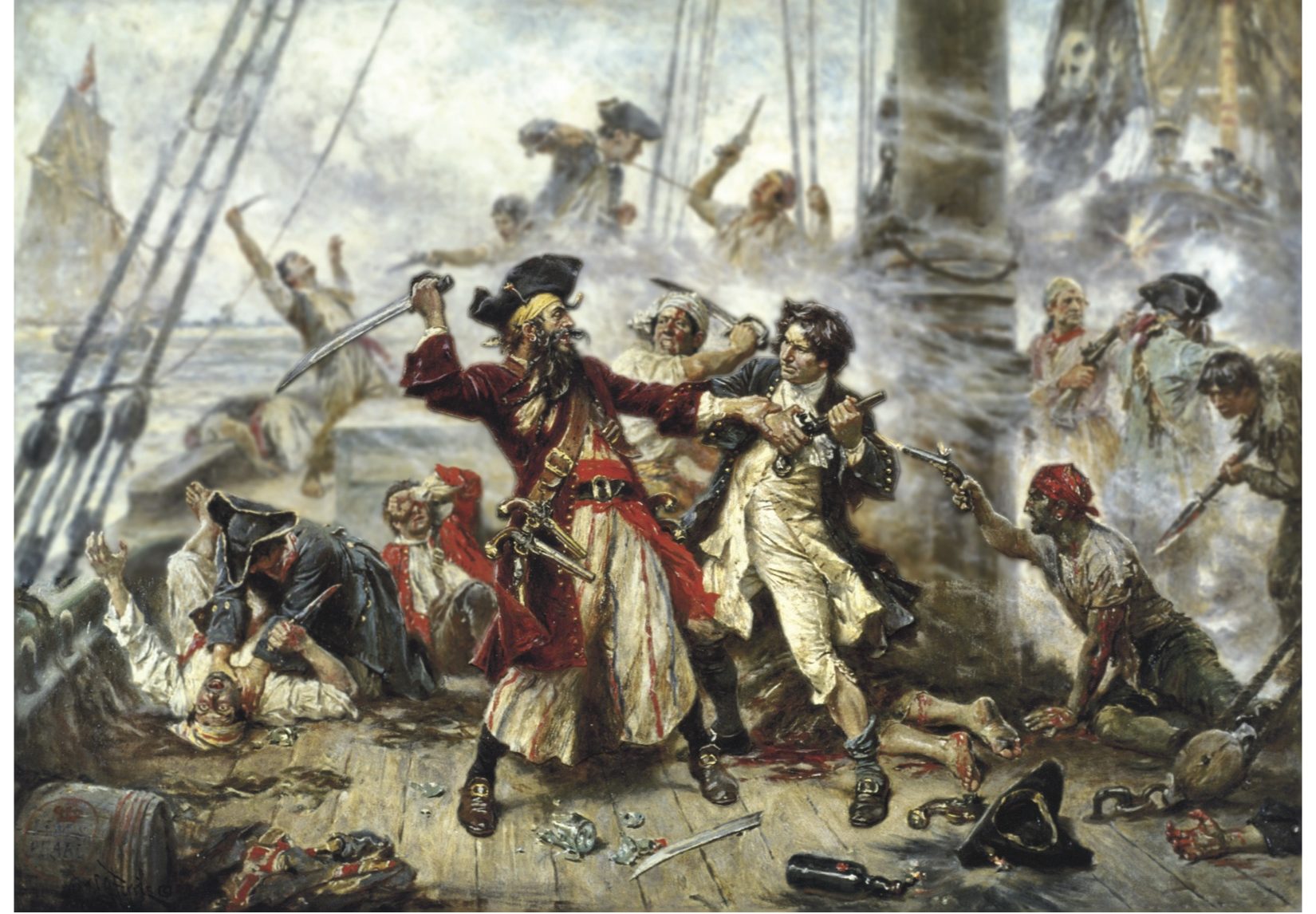The artwork captures an intense, chaotic battle scene aboard a large ship from the 1700s or 1800s, dominated by a vivid struggle between pirates and shipmates. In the foreground, a pirate, dressed in a red long coat with two pistols hanging from his strap, brandishes a long sword against a hero who is fiercely fighting back with a black pistol held in both hands. Surrounding them, other pirates and sailors are engaged in violent combat, with one pirate on the right leaning on the ground while firing a pistol, and another figure behind him wielding a rifle with a bayonet. The deck is strewn with swords, liquor bottles, and detritus, with smoke and seawater spraying all around, creating an atmosphere of chaos and desperation. The main mast of the ship is slightly visible towards the right, with a pirate flag prominently displayed, and the mast of another ship can be seen in the distance. Rope rigging and sail canvas frame the scene on the left, while the deck below is littered with fallen bodies. Smoke fills the air, obscuring the boundaries of the battle and heightening the sense of turmoil in the frame.